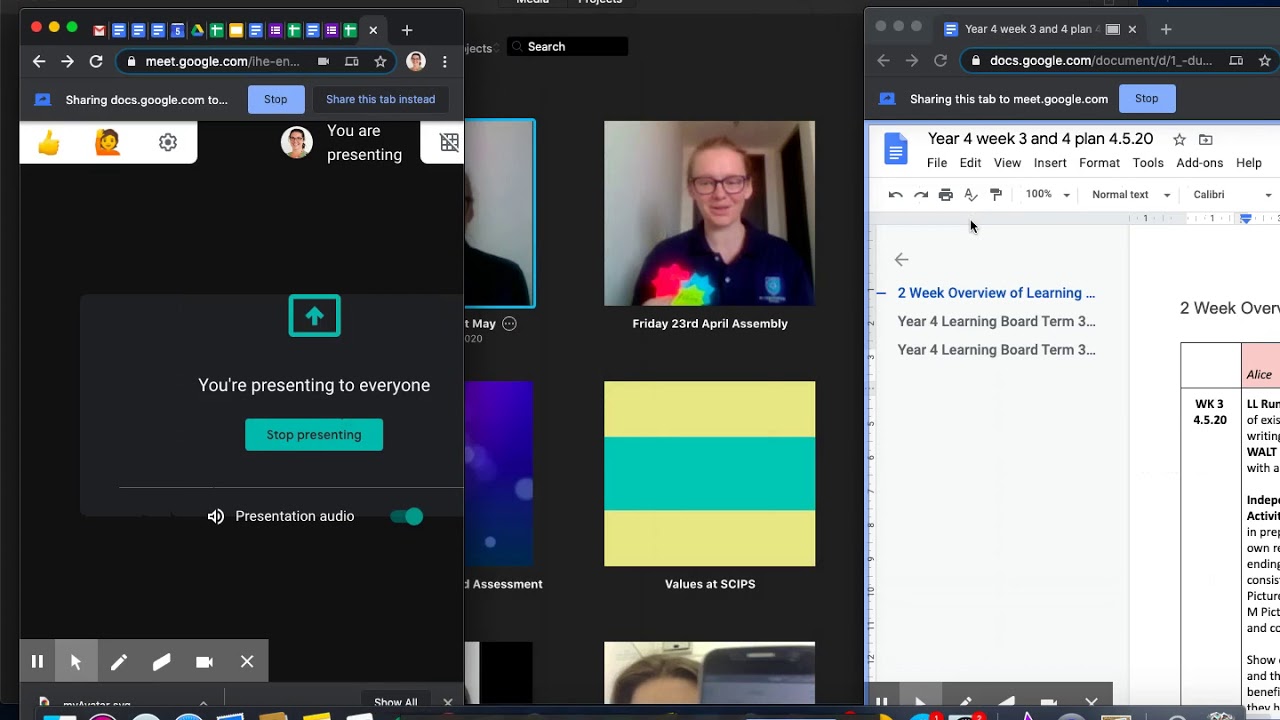A detailed description of the webpage presenting a Google Meet session:

The webpage depicts the interface of Google Meet, a platform not commonly familiar to the viewer. Situated in the upper corner is a notification displaying "You are presenting," accompanied by a thumbnail image of a woman. Beneath the thumbnail, text reads "Friday, April 23rd Assembly," followed by further information indicating "You're presenting to everyone." Adjacent to this notification is an upward arrow icon outlined in turquoise and a rectangular "Stop Presenting" button also in turquoise.

Scrolling down, control buttons for the microphone, which is currently enabled, are visible. Directly below the presenter's image, a distinct square icon is observable, featuring three horizontal stripes—where the outer stripes are yellow, and the middle stripe is turquoise. This symbol seemingly relates to a "Two-week overview of learning," hinting that the context might be within an academic setting.